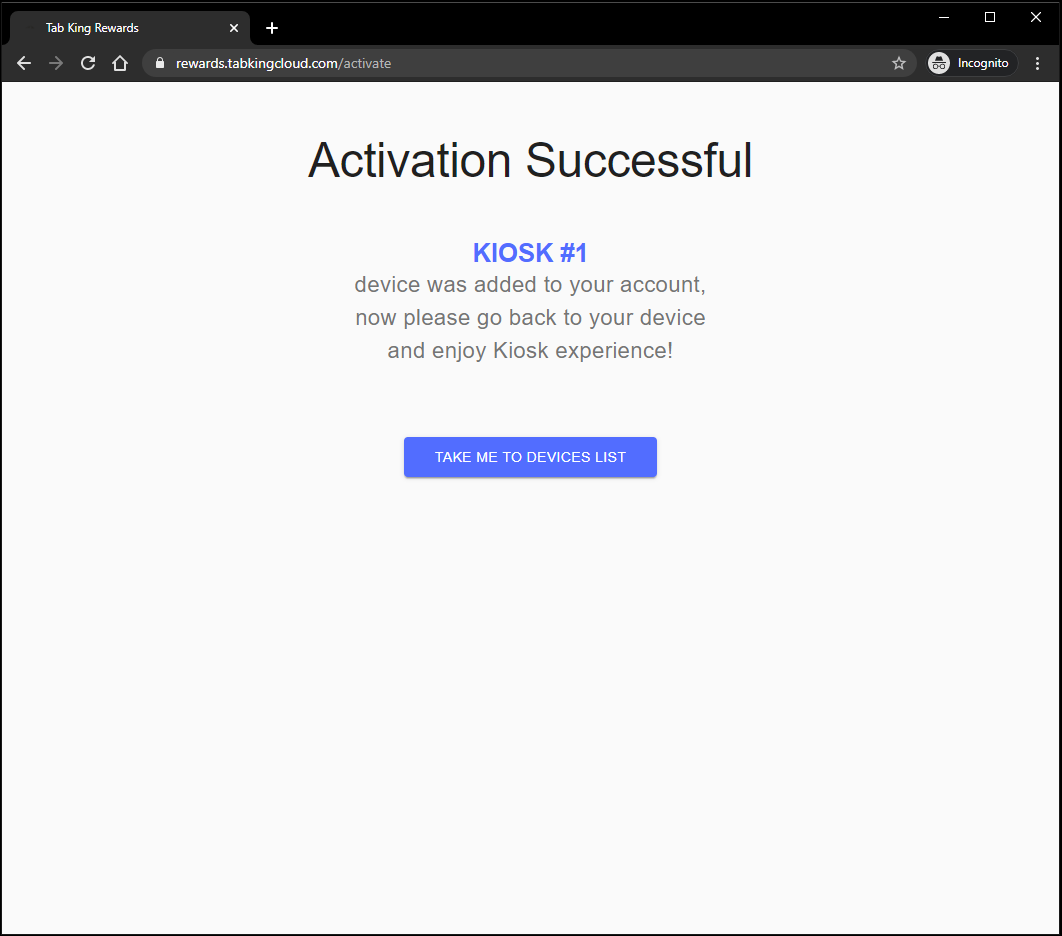The webpage features a sleek black header at the top, prominently displaying "TabKing Rewards" in white text, alongside a dark gray search bar. Positioned to the right, white icons of a minus sign, a square, and an 'x' are visible, beside another identical search bar. In the search bar, the URL "rewards.tabkingcloud.com/activate" is typed, accompanied by a lock icon that indicates a secure connection.

On the far right of the header, white icons for a star outline, an incognito icon labeled "Incognito," and a three-dot menu are present. Below the header, the background transitions to plain white, where a message in large black text reads "Activation Successful." Beneath this, in blue letters, the site designates "Kiosk Number 1" (spelled as "K-I-O-S-K Number 1"). A follow-up gray text informs the user that "Device was added to your account. Now please go back to your device and enjoy kiosk experience."

Further down, a distinctive blue banner features a white text link saying "Take me to device list." The remaining portion of the background remains white, and the entire webpage is bordered by thin black lines, giving it a clean and organized outline.